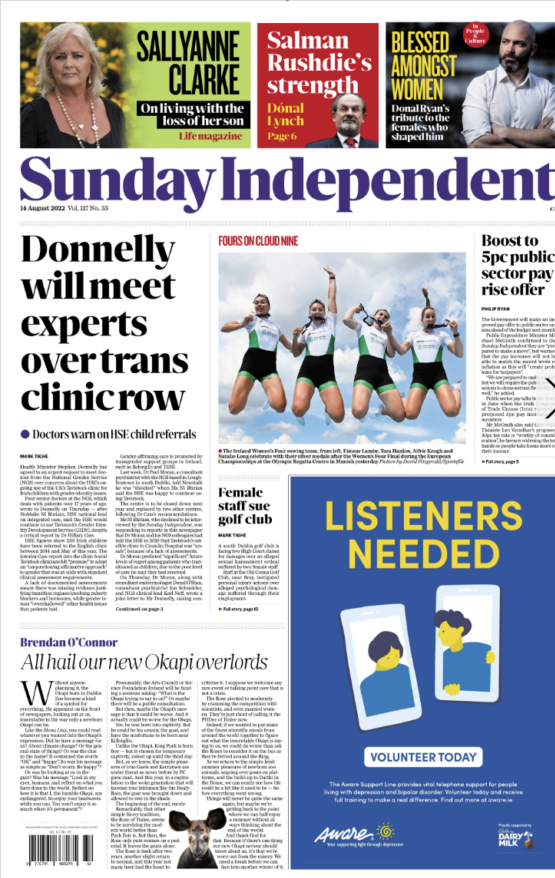This image showcases a screenshot of a newspaper front page. At the top, there are three prominent article headlines: "Sally Clark," "Salman Rashad," and "Blessed Among Women," indicating features on a woman, a man, and another person, possibly of revered status. Directly below these headlines, the masthead reads "Sunday Independent" in bold, dark lettering.

Beneath the masthead, a large article occupies the central area with a striking headline, written in bold, dark text. Adjacent to this article, there is an evocative image of a woman in mid-jump, hinting that she may be part of a sports team or athletic event. Alongside, there are smaller, illegible news articles filling out the rest of the layout.

At the bottom of the page, a large blue square features text in vibrant yellow: "LISTENERS NEEDED." This call to action encourages readers to "VOLUNTEER TODAY," accompanied by two cartoon images. Additionally, there is a humorous proclamation: "ALL HAIL OUR NEW OK API OVERLORDS," whimsically illustrated with a kangaroo-like figure. The bottom right corner includes a barcode, adding a final touch to this diverse and dynamic newspaper front page.